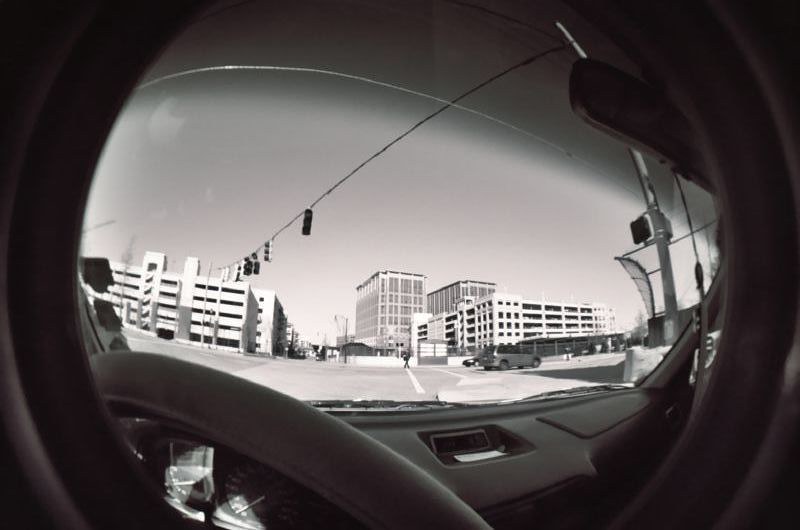The black and white photograph captures a city scene through the front windshield of a car, taken from the driver's perspective. The image forms a circular view, framed by a partially obstructed windshield that has a visible crack running through its upper part. Inside the vehicle, the gray dashboard and the top portion of the steering wheel are visible along with the speedometer. 

Outside, the car is stationary at an intersection. Ahead, the street is lined with concrete buildings; prominent among them are two tall, rectangular structures on either side—both resembling parking garages. Behind the building on the right, taller buildings loom in the background. The street is adorned with old-school style traffic lights hanging from a black rope attached to a silver pole at the corner.

The intersection is populated with a few vehicles; a silvery gray SUV is parked on the right side while another car is in the distance on the left, appearing to be in motion. A person is visible crossing the street. The sky overhead is mostly clear, with slight cloud formations discernible in the upper left corner of the image.